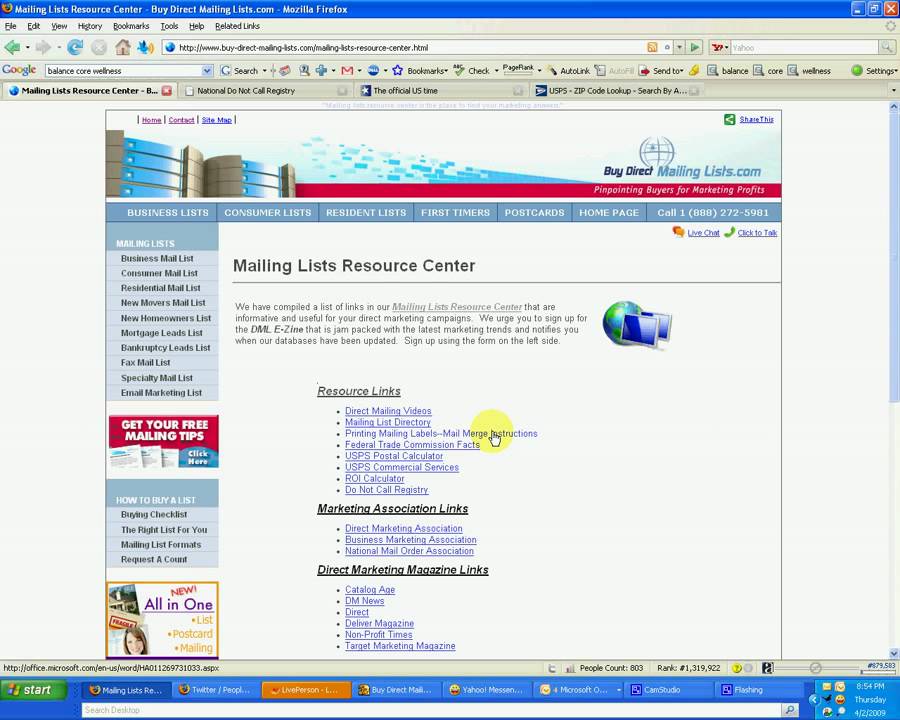A comprehensive view of the "Mailing Lists Resource Center" webpage by DirectMailingLists.com. The top navigation bar includes tabs for Home, Contact, and Sitemap. On the right, there is a "Share This" feature. Below "Share This," there's an image of an office building accompanied by the website's globe logo.

The main menu features several tabs: Business Lists, Consumer Lists, Resident Lists, First Timers, Postcards, Homepage, and Call - along with their contact phone number, 1-888-272-5981.

On the left section of the page, there are multiple selections, though the text is unclear. Centrally positioned is the headline "Mailing Lists Resource Center," followed by an introductory statement: "We have compiled a list of links in your Mailing Lists Resource Center."

To the right of this section is a small, unreadable text, with adjacent artwork depicting a globe and two computer monitors. Below these elements are various resource links categorized as follows:

1. **Resource Links**: Multiple unlabeled links.
2. **Marketing Association Links**: Three specific links.
3. **Direct Marketing Magazine Links**: Eight individual links.

This detailed structure provides a practical interface for users seeking a wide array of mailing list resources.